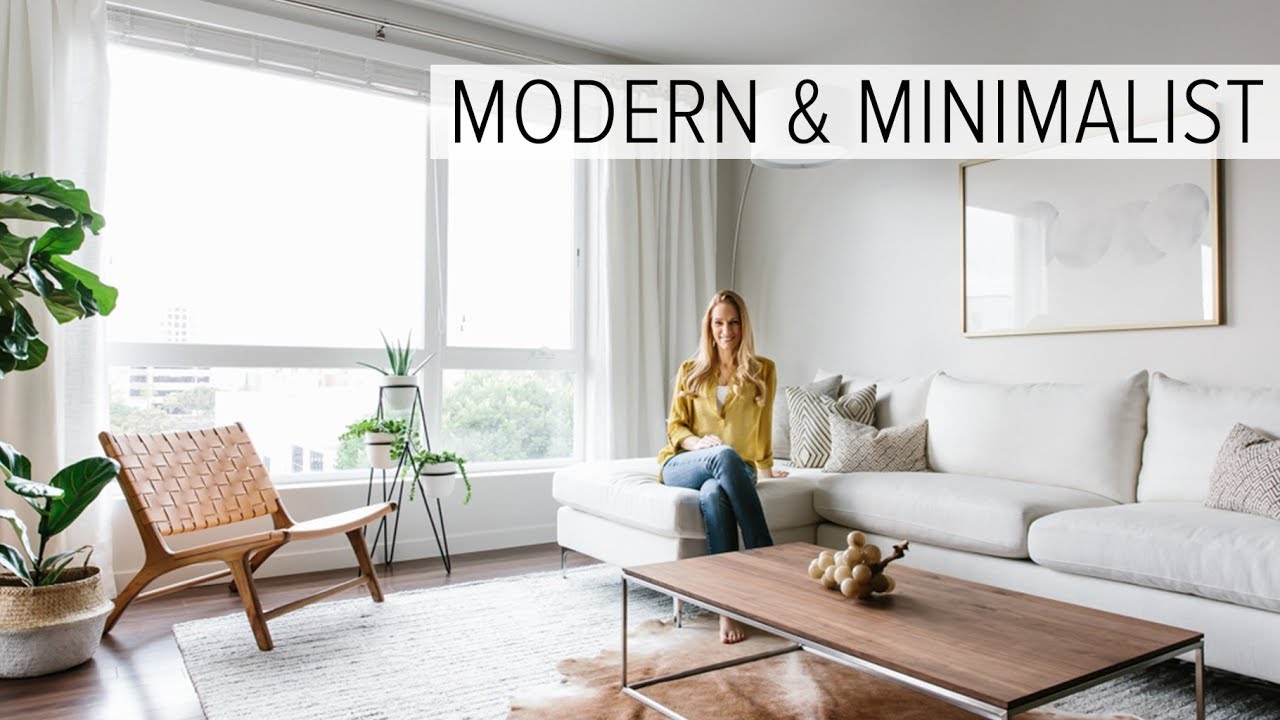In the contemporary and minimalist living room, a smiling blonde woman sits comfortably on a white couch. She is dressed in a yellow blouse over a white camisole, paired with light blue jeans. The room features white walls decorated with a minimalist art piece in a golden frame, showcasing simple grey blotches. Above the art piece, a text banner reads "Modern and Minimalist." To her left, a large window with white curtains and a cross divider lets in natural light, somewhat veiling the view of the city outside. The room also includes a woven wooden chair, a wooden coffee table with chrome legs, and a white rug with brown and red gradients. Simple patterned pillows adorn the couch, and there's a potted plant with large leaves in the corner and another beside the chair, enhancing the serene ambiance. Overall, the decor is simple yet elegant, reflecting modern minimalist aesthetics.